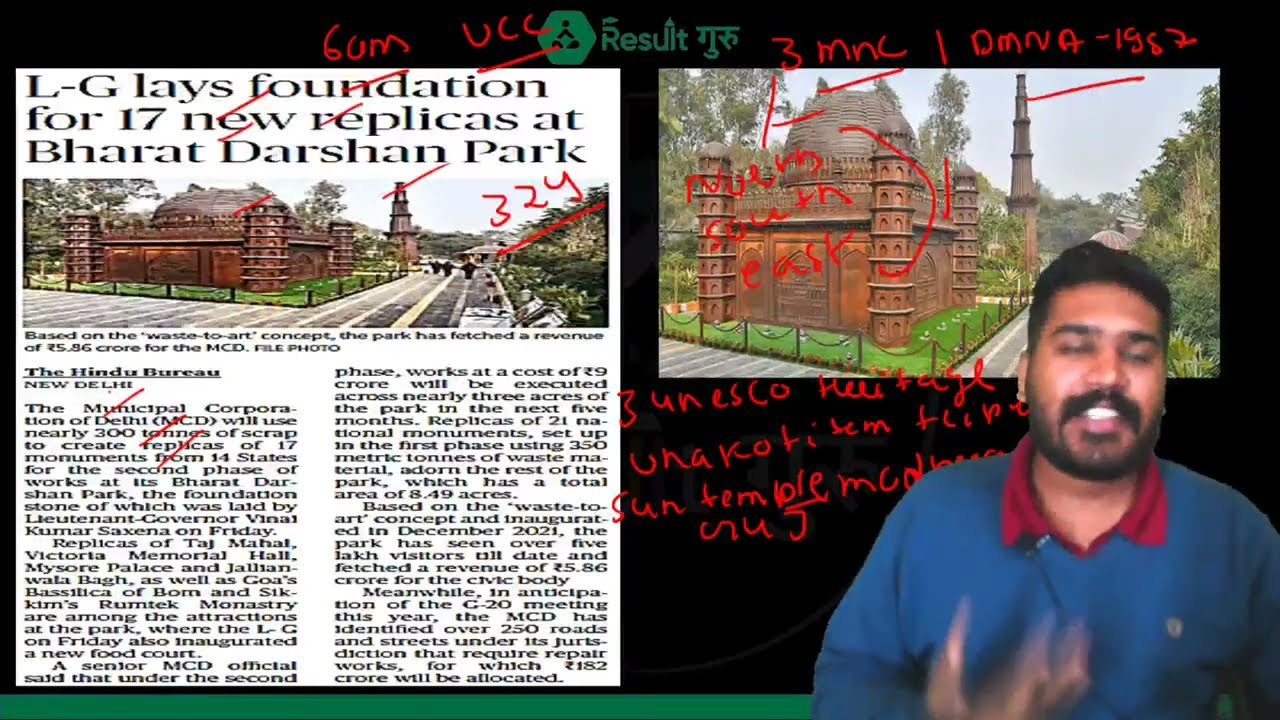The image features a motion-blurred photograph of a Hispanic man with dark black hair, longer on the top than the sides, and a full beard. He is dressed in a blue shirt with a maroon collar, and his mouth is open, revealing shining teeth. His hand is raised above his chest with fingers streaking upwards due to the blur. He is positioned in front of a black background adorned with two superimposed images and red handwritten annotations. 

To his left, a newspaper article titled "L-G lays foundation for 17 new replicas at Bahat Darshan Park" is visible. The article details the park's development, highlighting its waste-to-art concept, which has generated significant revenue for the Municipal Corporation of Delhi. Below the title, there's an image of a brown castle with round columns, surrounded by greenery and a rope barrier. Text underneath describes the park's features and future plans, mentioning various replicas and the inauguration of a new food court. Additionally, an official cited that the park will expand using 300 tons of scrap to create 17 monuments in the second phase, among other details. 

On the right side, the background features another image of the same brown castle and lush trees, reinforcing the theme of the article. The detailed annotations and visuals create a composite backstory, merging the man’s blurred, animated presence with the historical and cultural narrative of the Bahat Darshan Park’s monumental replicas.